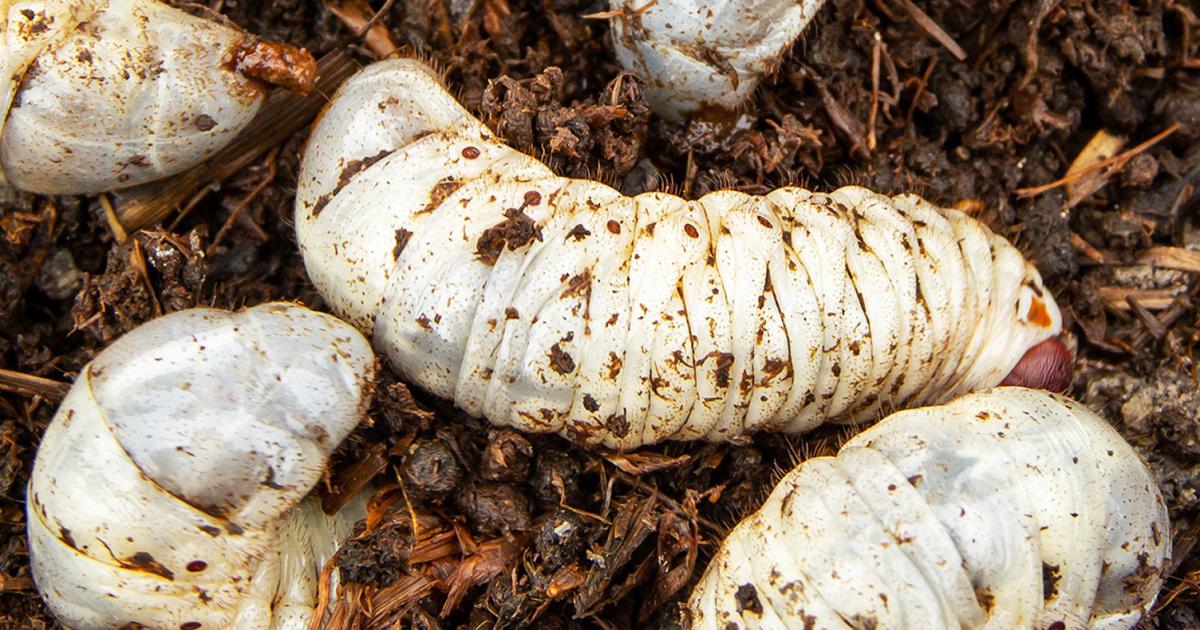This is a high-resolution, close-up photograph of five white grubs situated within a moist, brown dirt and mulch environment. The image, captured with significant clarity, reveals intricate details such as small twigs and clumps of dirt scattered amongst the grubs. The fully visible central grub is distinct, while the other four are partially seen: one revealing its tail end at the upper left, another partially burrowed at the bottom left, one with just its top part visible at the bottom right, and the last showing part of its head at the top center. The grubs exhibit various shades, with some areas appearing grayish and others pinkish. The photograph is free of any text and likely taken during daylight, emphasizing the natural outdoor setting.